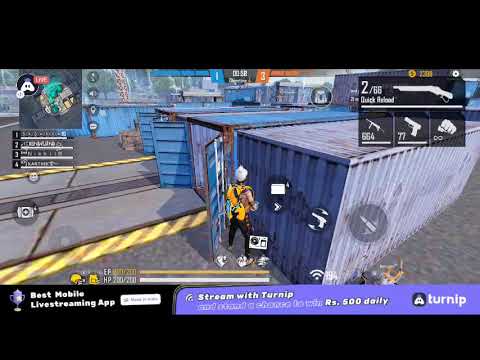The image appears to be a screenshot from a third-person shooter video game. It features a character standing outdoors near metallic, rectangular storage containers typically used for shipping. One container is rusty blue, and the other is silver. The character, who is somewhat blurry, is wearing a yellow vest, dark pants, and a white hat. He appears to be holding a weapon, possibly a rifle. 

In the bottom left corner of the image, there is text stating "Best Mobile Live Streaming App" alongside a small purple trophy. It also reads "Stream with Turnip, RS500 Daily." The bottom right corner displays the word "Turnip" in white font, suggesting another reference to the streaming app. 

In the top left corner, there is a map providing an aerial view and displaying the character's current location. Additionally, a leaderboard numbered one through four is present. On the right side of the image, there is a weapons panel showing various options including a shotgun, machine gun, pistol, and the option for hand-to-hand combat (denoted by a fist icon). The ammo count for the selected weapon and the infinite punching ability are also displayed.